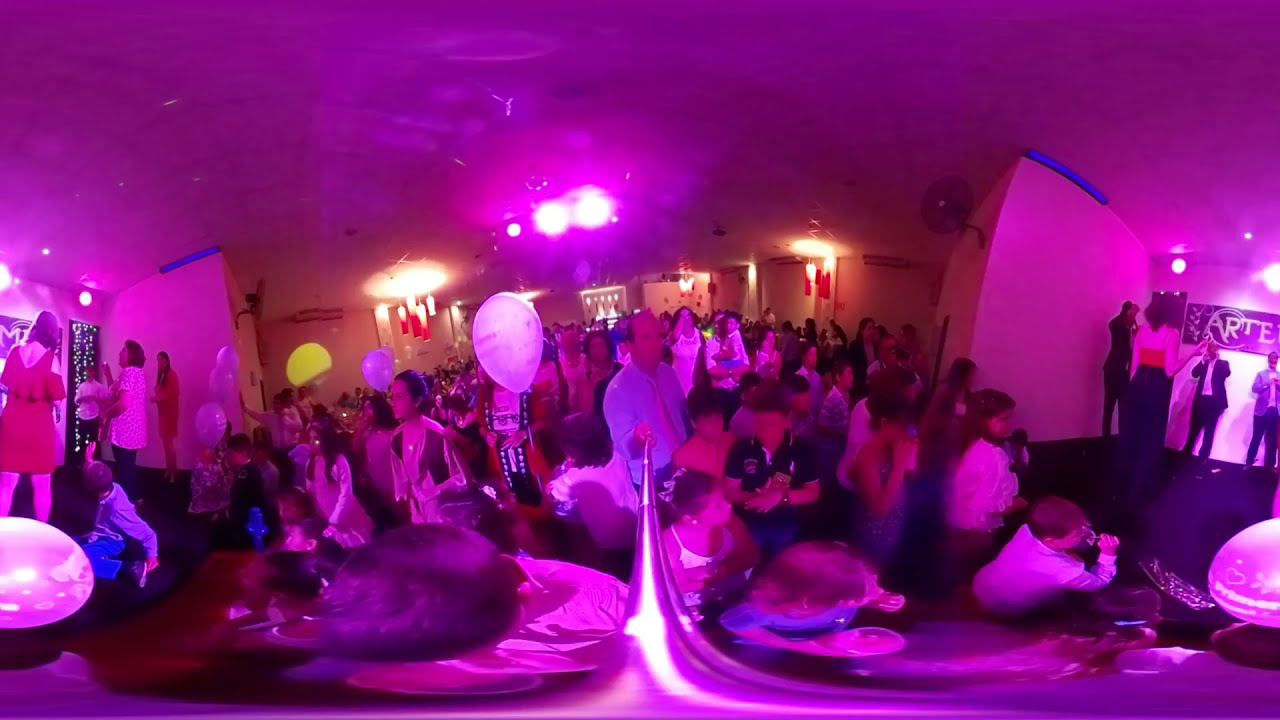The image is a fisheye lens panoramic photograph capturing a lively indoor celebration, with the entire scene bathed in a vibrant purple-pink hue, likely from overhead circular lights. At the center, a man with a receding hairline, dressed in a light blue shirt and tie, is taking a selfie using a selfie stick. The stick is visible, pointing towards the bottom center of the image. The room is crowded with people, many dressed in white, though there are splashes of other colors, including two women in red dresses. Balloons add to the festive atmosphere. The scene includes what appear to be stages on both the left and right sides, possibly hosting performances. There are also fans and blue lights mounted on the ceiling, enhancing the celebratory ambiance.